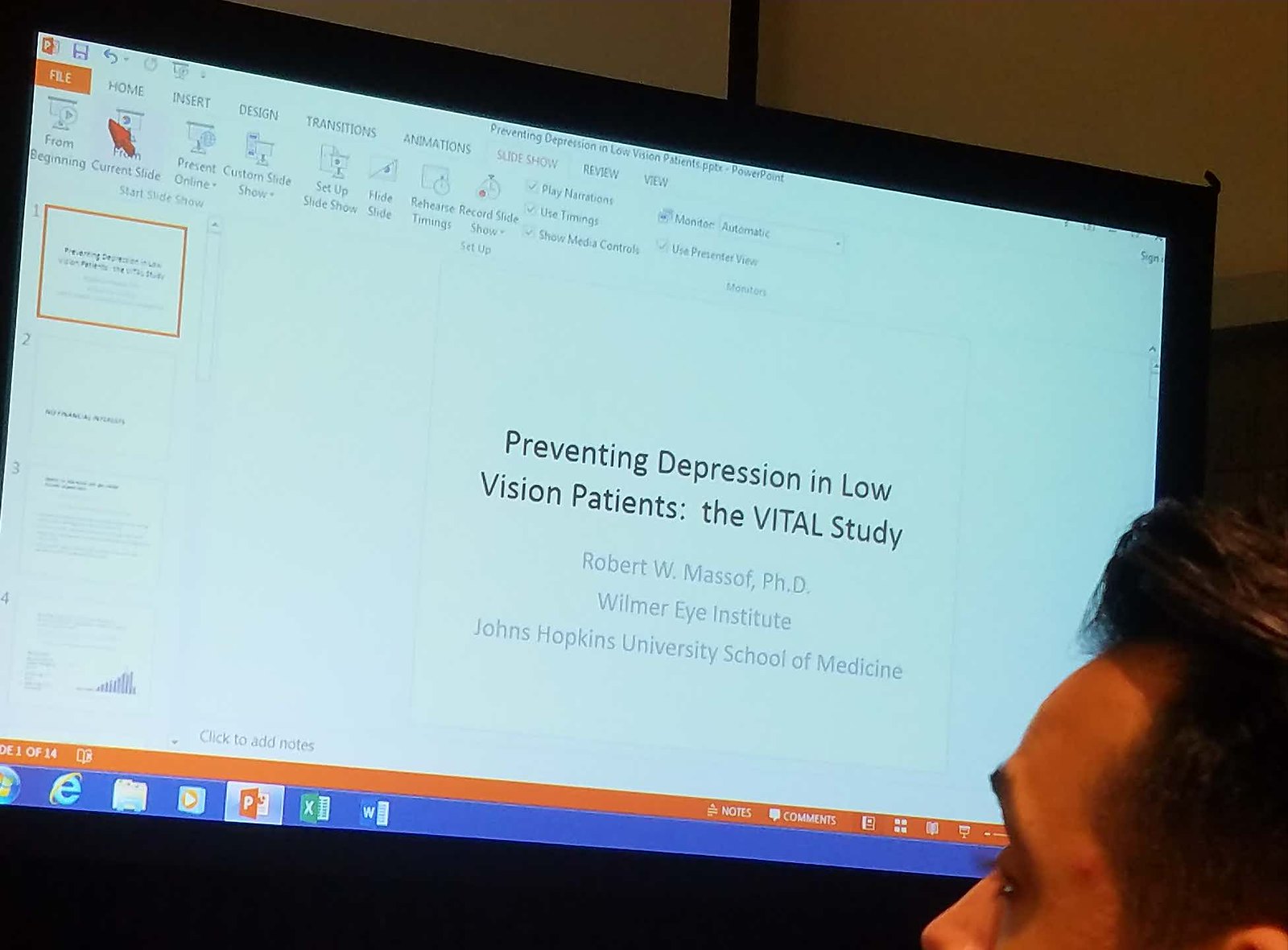The photograph, taken indoors, is a rectangular image roughly six inches wide and five inches tall. Dominating the scene, a young man with short brown hair and a pointed brow is visible in the lower right corner, his upper left profile illuminated. Due to the lighting, his skin appears orange, highlighting a small pimple on his temple. His gaze is fixed upward toward a large TV or computer screen framed in black.

The screen displays a white background with black text prominently featuring the title, "Preventing Depression in Low Vision Patients, The Vital Study." Additional text on the screen credits Robert W. Massa, Ph.D., Wilmer Eye Institute, John Hopkins University School of Medicine. The screen is clearly a PowerPoint presentation, evident from the editing tools at the top. Words such as "File," "Home," "Insert," "Design," "Transition," and "Animations" are visible, with "File" highlighted in orange and the orange mouse pointer directed towards it. The darkened wall behind the screen is partially visible in the upper right corner of the image. The detailed editing bar on the screen shows an orange top section and a blue bottom section, indicating this is a work in progress, presumably one of 14 pages, possibly being finalized in an office environment.